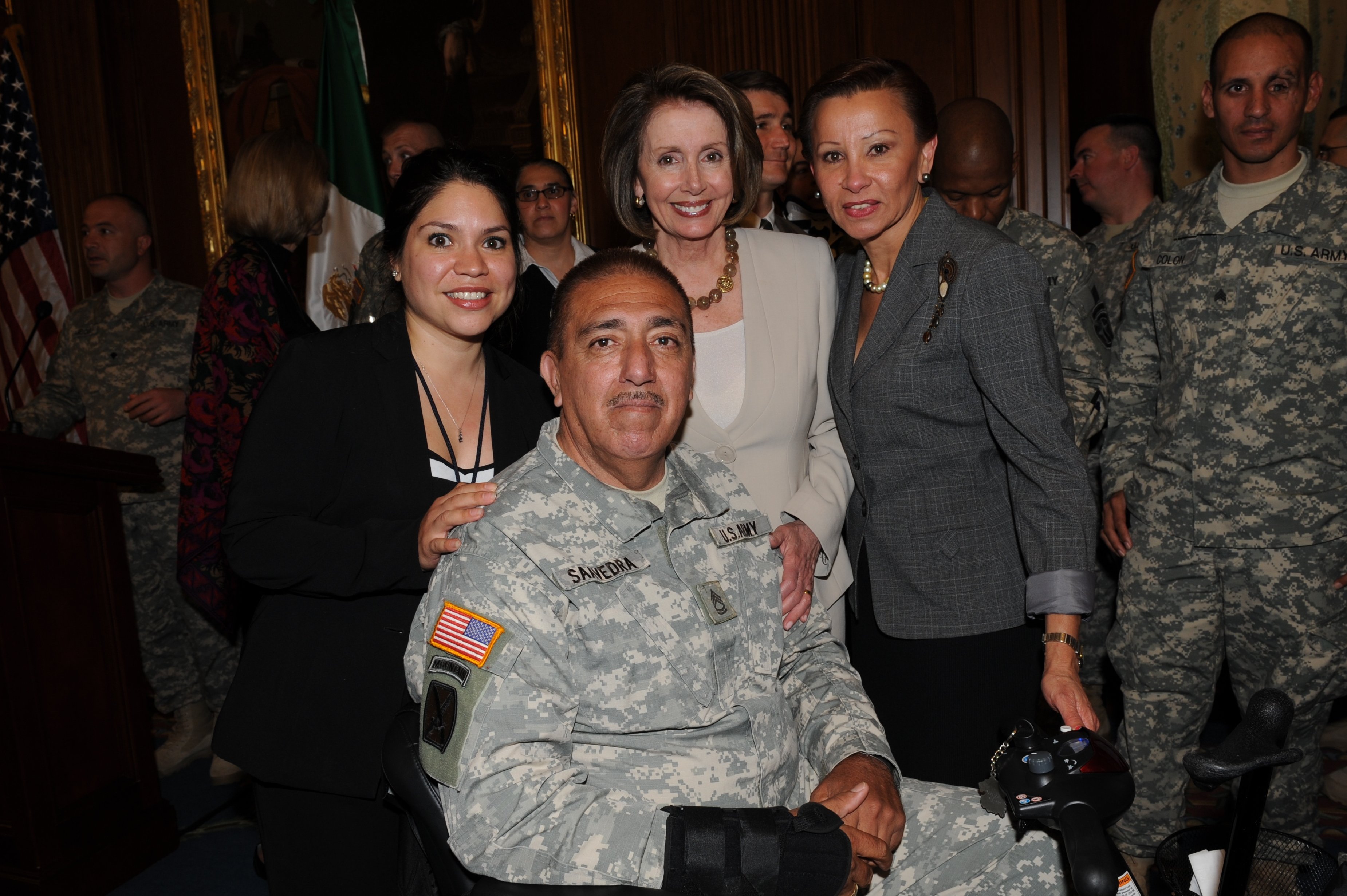The image portrays an intimate indoor gathering featuring a diverse group of individuals. Dominating the foreground is a seated man with tanned skin, dressed in military fatigues, identified with the name "SAVEDRA" and "U.S. Army" on his uniform. He has a serious expression and appears to be wearing a wrist support on his right hand. Standing directly behind him to the left is a woman with dark hair tied back, wearing a black suit jacket over a black and white top, smiling warmly at the camera. 

To the right of her stands another woman recognized as Nancy Pelosi, distinguished by her mid-length dark hair, a white top paired with a greyish-beige blazer, and a prominent chunky necklace. Adjacent to Pelosi is another woman with short brown hair, clad in a grey jacket and black trousers. Further to the right, there is another individual in military attire, and the background reveals an assorted mix of additional people, some dressed casually and others in varied military uniforms. The scene captures the intersection of civilian and military individuals, encapsulating a moment of shared presence and camaraderie.